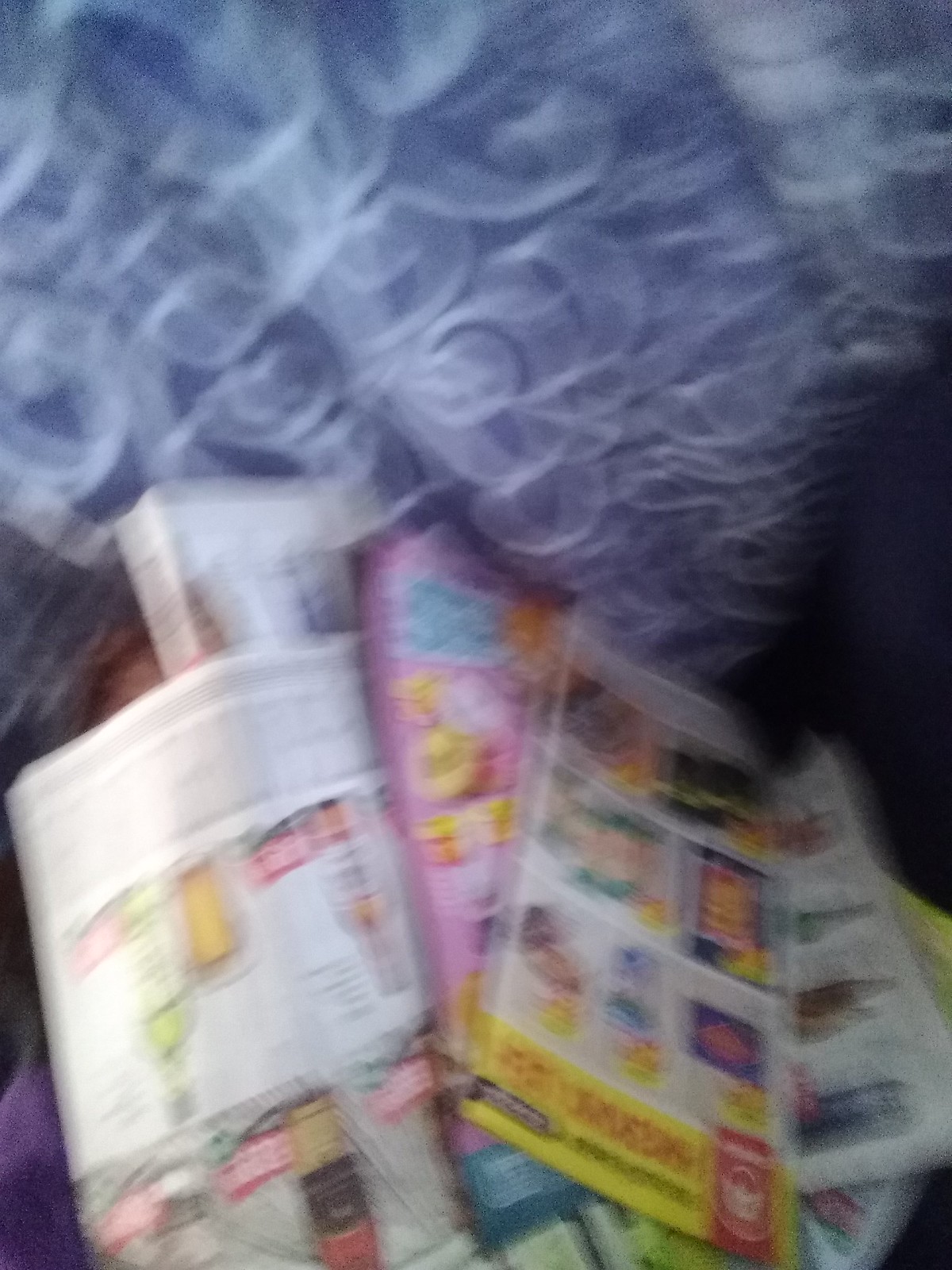The image portrays a very blurry scene featuring a pile of magazines or advertisements on a white and blue fabric background with swirling, smoky-like patterns. The fabric occupies the top of the picture, characterized by its navy-blue base and flowing white swirls that resemble smoke but are not actual smoke. Beneath this fabric background, we see a stack of various colorful pages, likely advertisements or sales inserts, aligned upside down with their tops towards the bottom of the image. The topmost item in the stack has a yellow label and features a series of eight different product pictures, including chips and a can. Below this, there is a pink square advertisement, possibly targeted at women or young girls. Further down, there appears to be a magazine-like insert, likely advertising wines, though the details are blurry. Additionally, a hint of a blue-colored insert can be seen beneath the pile. In a small section towards the left, the top right corner of someone’s forehead and the bottom left possibly a right shoulder in a purple shirt appear faintly, adding to the overall indistinct and hazy appearance of the image.